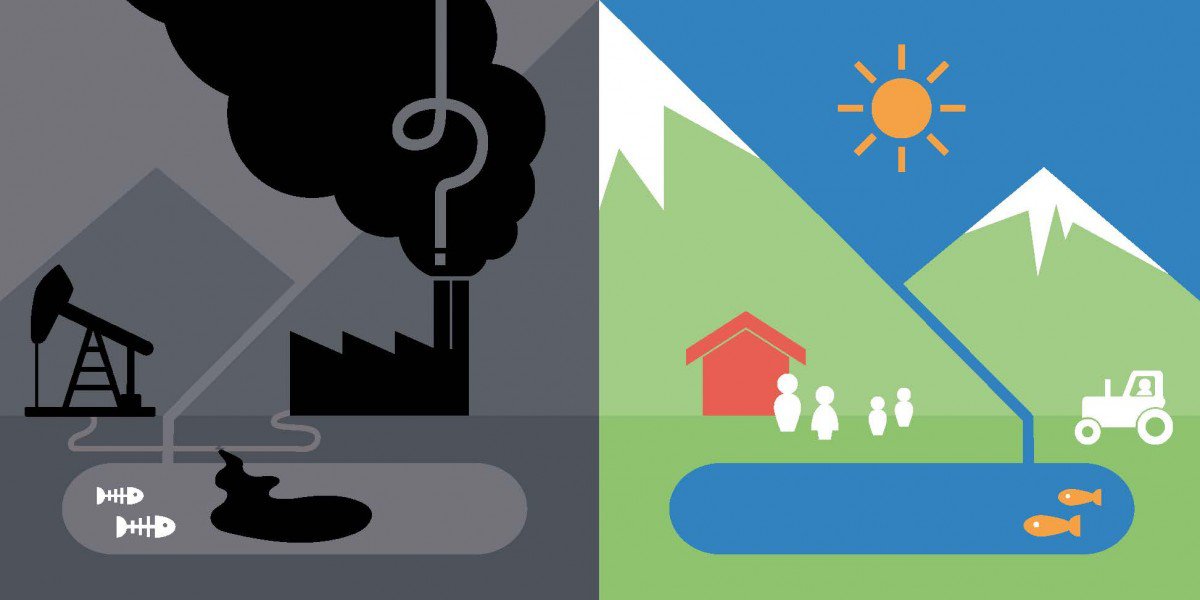This illustrated rectangular image is divided into two contrasting halves. In the center of the image stands a mountain, which is split to reveal two distinct scenes. The left side depicts a dark, gloomy environment dominated by industrial activities. A silhouette of a factory emits black smoke against the backdrop of gray mountains. An oil drilling rig is seen near a contaminated lake, where oil spills have turned the water murky and left behind fish skeletons. The overall atmosphere is bleak and depressing.

Contrasting sharply, the right side of the image is bright and cheerful, bathed in sunlight. Here, the mountains are green with snow-capped peaks under a clear blue sky, where a radiant sun with eight rays shines down. A vibrant blue lake houses two living, orange fish with white eyes. Nearby stands a red farmhouse with four people—a man, a woman, and two children—enjoying the serene setting. A white tractor is situated to the right of the house, enhancing the peaceful and idyllic scene.

Overall, the image starkly contrasts the dismal effects of industrial pollution with a picturesque, harmonious rural landscape.